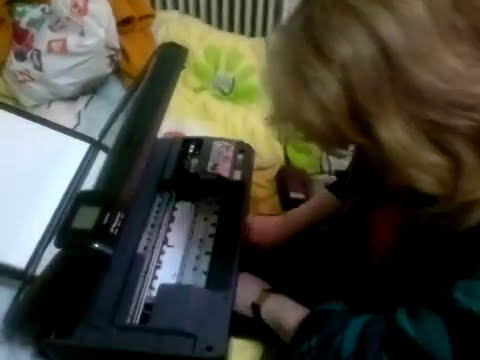In this detailed color photograph, a Caucasian woman with long blonde hair is seen attempting to repair a sizeable, bulky black printer, which appears to be a model from the 2000s. The printer's top is open, revealing its internal mechanisms including a glass screen and silver metal parts, indicating she is likely addressing an issue inside. Positioned predominantly on the right side of the frame, the woman is seated on what seems to be a bed, adorned with yellow pillows, floral-patterned blankets, and other bedclothes. She wears a dark green shirt with sleeves pushed up, and a wristwatch on her left hand is visible. Her hands are engaged with the inner components of the printer, which is directly in front of her, slightly to the left. Additionally, a white plastic shopping bag with contents is noticeable in the upper left corner of the image, alongside a white radiator and an orange garment. The ambient setting, coupled with her focused attention on the printer, suggests she's troubleshooting a technical issue with the device.